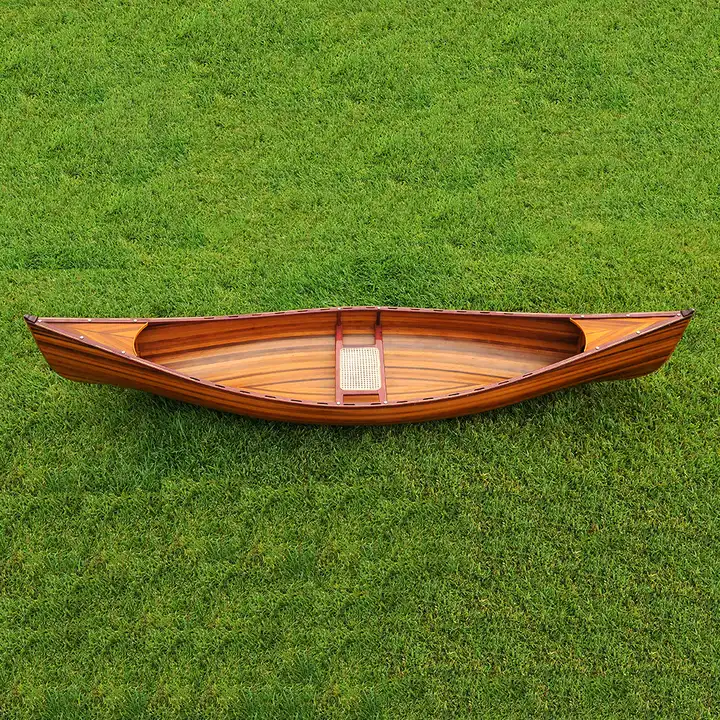This overhead photograph captures a newly crafted, wooden canoe elegantly centered on a lush, meticulously manicured lawn. The vibrant green grass provides a picturesque backdrop, framing the canoe with its smooth and carefully maintained surface. The canoe is small, likely built for a single person, and showcases a harmonious blend of craftsmanship and natural aesthetics.

The canoe itself features symmetrical yellow and red alternating boards along its length, equipped with a seat positioned in the exact center. This seat consists of a wooden frame supporting a center made of white woven material, possibly cane, adding to the traditional look. The wood is polished to a high sheen, reflecting its recent construction, though the overcast sky minimizes any glaring reflections.

Around the canoe's perimeter, a wood border is punctuated with visible screw heads or rivets, hinting at the meticulous attention to detail in its creation. Both ends of the canoe taper to sharp points, maintaining a classic canoe form while the slight flat areas at the tips emphasize its balanced design. The absence of clear signs indicating a front or back reinforces the symmetrical nature of this beautifully crafted vessel.